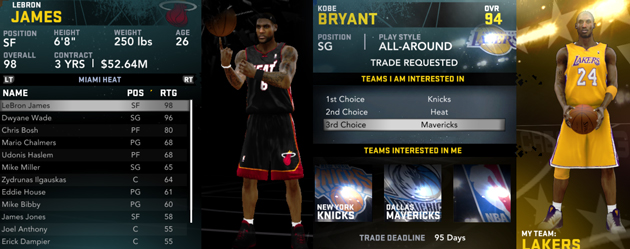This image is a screenshot from a basketball video game, featuring player statistics for two iconic NBA players. On the left, LeBron James is detailed with an overall rating of 98. He plays the Small Forward (SF) position, stands at 6'8", weighs 250 pounds, and is 26 years old. He has a contract of 3 years for a total of $52.64 million.

On the right, Kobe Bryant is highlighted with an overall rating of 94, primarily playing as a Shooting Guard (SG) with an all-around play style. Notably, he has requested a trade from his current team, the Lakers. His top three preferred destinations are the New York Knicks, Miami Heat, and Dallas Mavericks. The trade deadline is set at 95 days. The screenshot captures key career details and stats for both players, providing a comprehensive comparison. Transcribed by https://otter.ai.